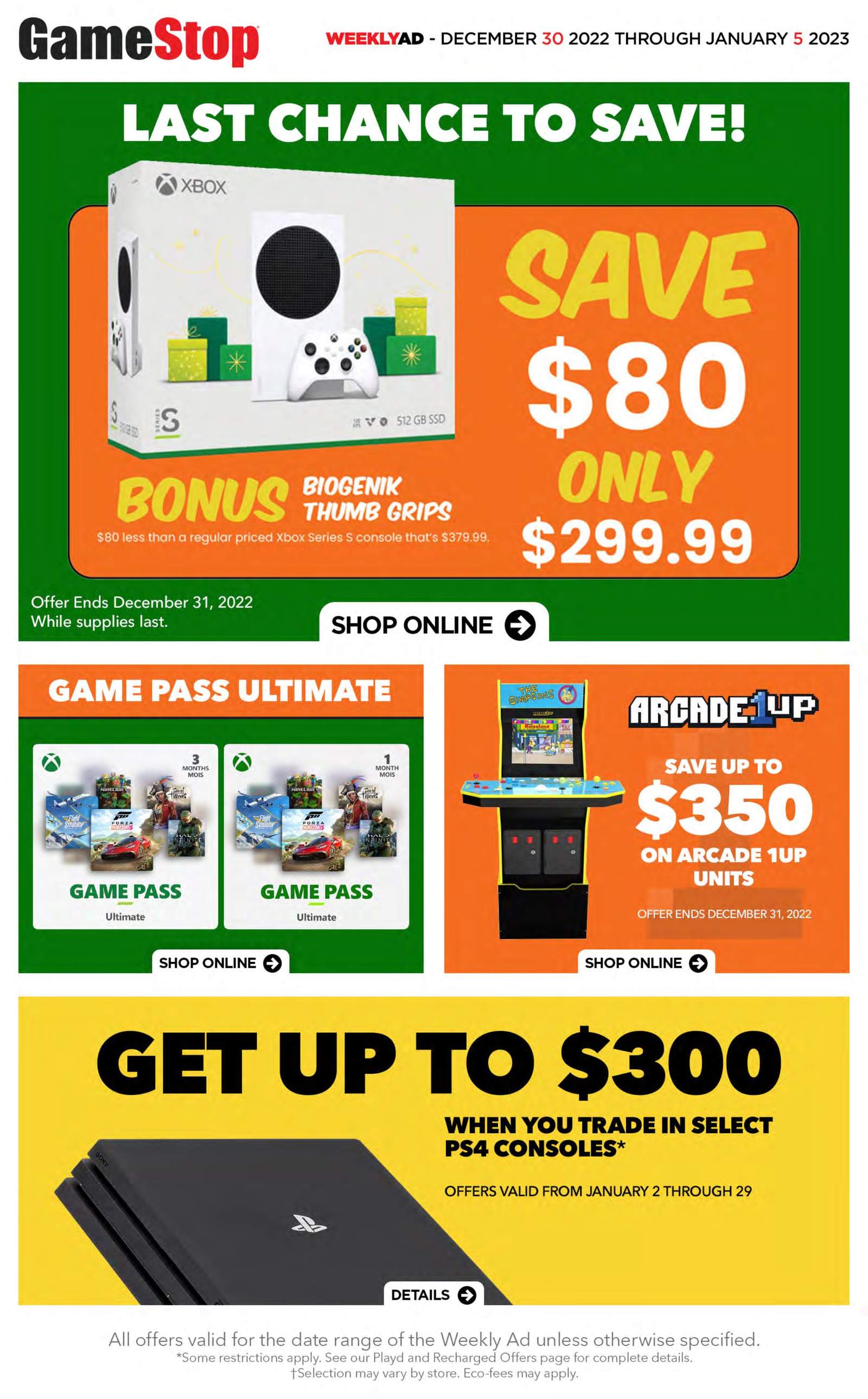This detailed caption describes a promotional web page for GameStop:

"This web page from GameStop features a header where 'Game' is written in black and 'Stop' in red, indicating the retailer's branding. The central section promotes their weekly ad running from December 30th, 2022, to January 5th, 2023. A prominent green rectangle highlights a 'Last Chance to Save,' offering an $80 savings with a bonus Biogenic Thumb Grip, priced at $2,999. Below this, the advertisement pushes for online shopping. Additionally, there's a section for 'Game Pass Ultimate,' showcased through two small square advertisements. Another promotional highlight features Arcade 1-Up units with potential savings of up to $350, each accompanied by an online shopping arrow icon. The page also mentions a trade-in offer, where customers can receive up to $300 for selected PS4 consoles."